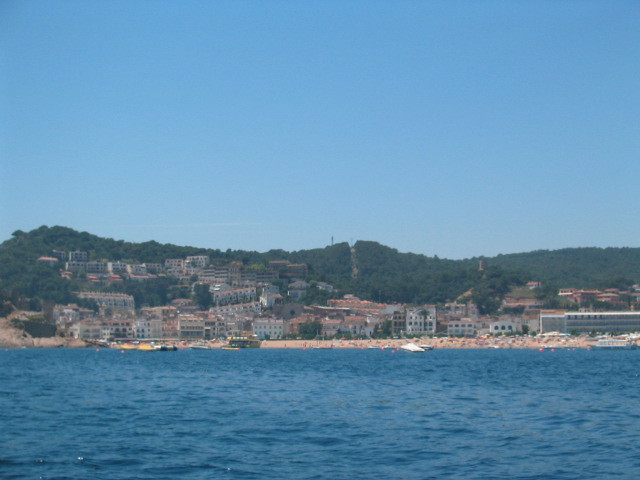The image captures a picturesque coastal village nestled against the side of a broad hill. At the bottom of the image, a large body of rippling, vibrant blue water stretches up to a sandy beach bustling with people. A couple of boats are scattered across the water, adding to the lively seaside atmosphere. The beach forms a clear, expansive line separating the water from the land. Above the beach, numerous residential buildings climb the hill, many of which feature multiple floors and rows of windows, predominantly concentrating towards the left side. The hill itself is lush and green with trees and shrubbery, indicating a rich, natural environment. Dominating the top half of the image is a bright, clear blue sky, flawlessly devoid of clouds, suggesting it's taken in the middle of a sunny day. The harmonious blend of water, land, and sky, with the village at the center, creates a serene and inviting outdoor scene.